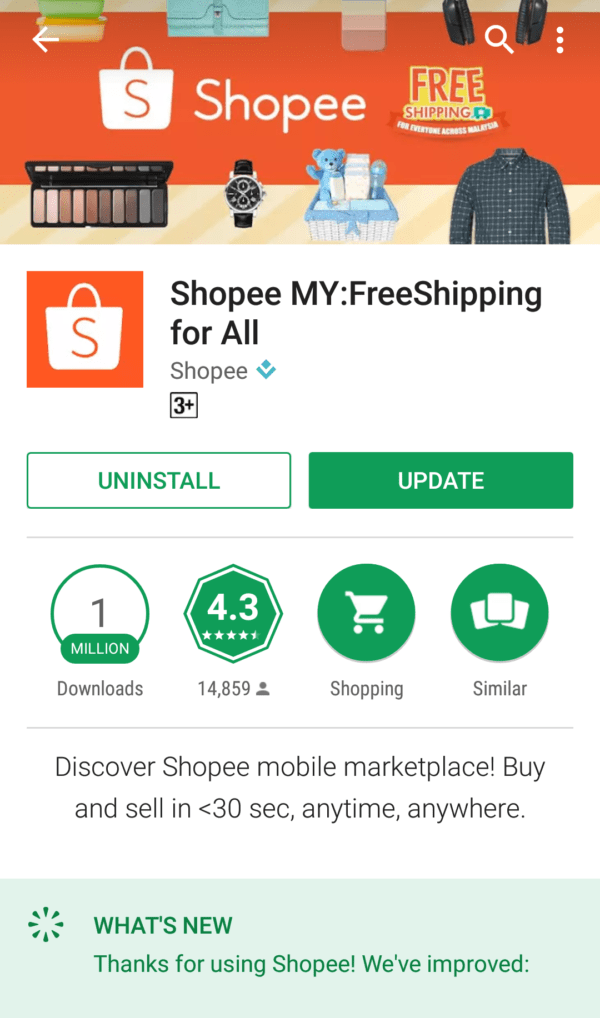This is a detailed and organized description of an image captured from a mobile shopping app called Shopee:

The image is a screenshot taken from the Shopee mobile app on a smartphone. At the top of the screen, there's an orange background setting a vibrant tone. Various items are displayed prominently, including a shirt, a baby gift set, a wristwatch, makeup products, and a bag marked with a large capital letter 'S'. Hanging in the background are additional miscellaneous items.

The text "free shipping" is displayed, highlighting a promotional offer. The bag prominently branded with the letter 'S' reinforces the branding of Shopee, spelled out as "S-H-O-P-E-E". Further down, the screen reads "Shop E, my" followed by the statement "free shipping for all". It also mentions "three plus in a box", indicating perhaps a special deal or set.

Below this section, there is an interactive area where users can choose to either "uninstall" or "update" the app, with the options presented in a white box with green text and a green box with white text, respectively.

Continuing down, there are four icons in the center: one indicating "one million downloads", another showing "4.3 stars" for user reviews, a "shopping" icon with a grocery cart, and an option labeled "similar". Additionally, a promotional tagline reads "Discover Shopee mobile marketplace. Buy and sell in less than 30 seconds, anytime, anywhere."

The clean design and emphasized promotional content showcase the ease and convenience of using the Shopee app for online shopping.